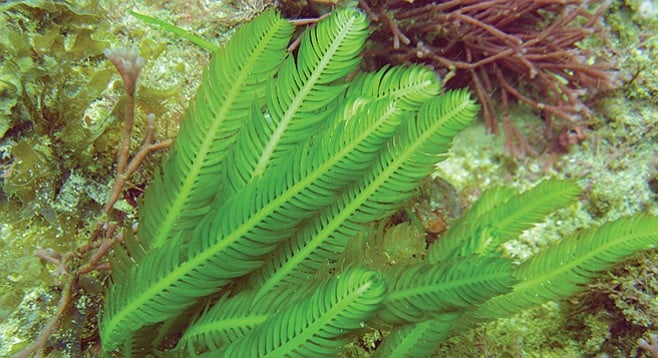A captivating underwater photograph featuring vibrant green feather-like algae, known as green feather algae, dominates the scene. These algae, resembling long, delicate millipedes with numerous thin leaves extending from each side of their long stalks, present a striking contrast to the other flora. Surrounding them are various other plant life, including some dark pinkish-brown and somewhat dead-looking plants laying flat against the whiteish ground. Additionally, there are sparse patches of dark pinkish-brown and light auburn vegetation. Although the background beyond the plants is not visible, there is a distinct underwater ambiance with no signs of rocks, shells, or fish. The photo captures only the lush aquatic plants, emphasizing their vibrant and diverse forms.